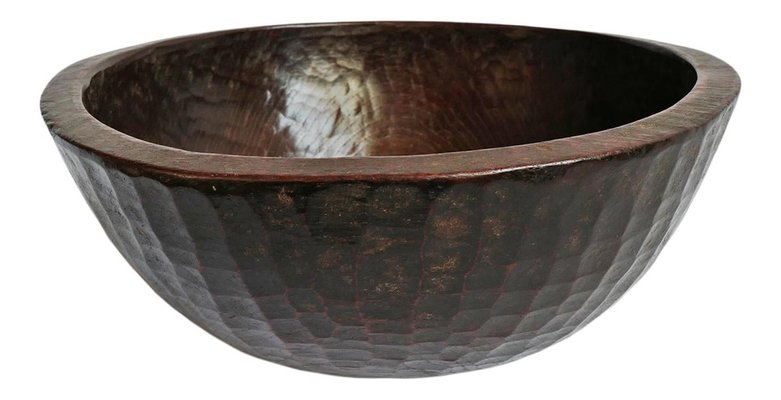This photograph features a rustic, brown wooden bowl set against an entirely white background. The bowl boasts a unique texture on its exterior that resembles the intricate patterning of tortoise or crocodile skin, giving it a distinct and appealing look. The dome-shaped structure is shiny on the outside, though not as much as the smoother interior, which visibly reflects light. The bowl shows signs of age, with noticeable wear and tear around the rim, including chipped and rubbed-off sections, especially on the far left and center right. These characteristics, combined with its patina, contribute to the bowl's vintage charm, enhancing its stylish and well-crafted appearance.